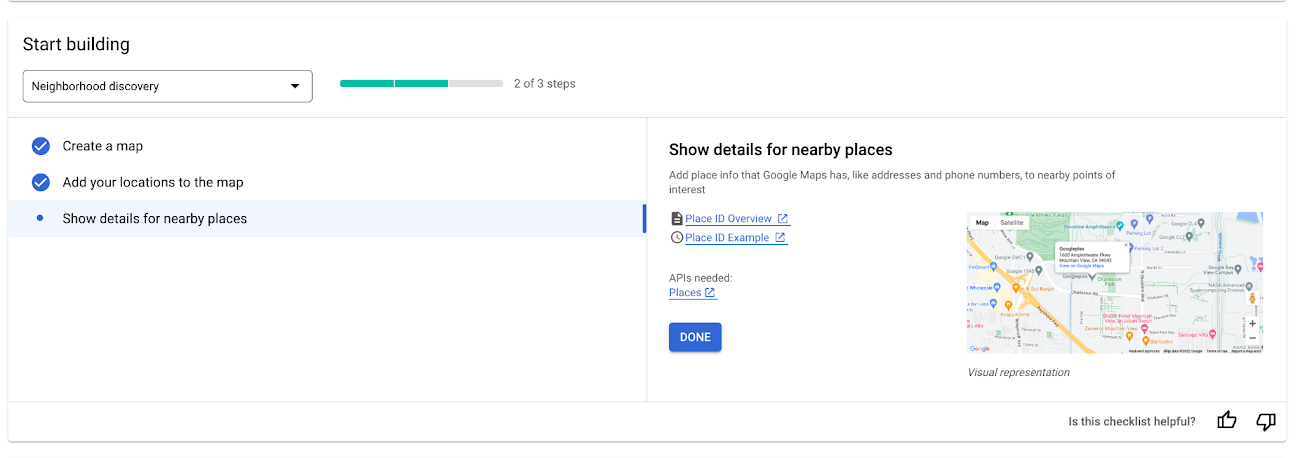This is a detailed description of a screenshot taken from a Google Maps personalization map. The image features a white background and is rectangular in shape. In the top left corner, bold black text reads "Start Building." Directly below this text is a drop-down box set to "Neighborhood Discovery." To the right of this drop-down box, there are three small horizontal lines; the left and center lines are green, indicating completion, while the right line is gray, denoting an incomplete step. Adjacent to these lines, the text reads "2 of 3 steps," signifying that two out of the three steps have been completed.

On the left side of the screenshot is a vertical list of three tasks. The first task, labeled "Create a map," is written in small black letters and is marked with a blue circle containing a white check mark. The second task, "Add your locations to the map," also has a blue circle with a white check mark, indicating completion. The third task, "Show details for nearby places," is highlighted with a blue line and is marked by a blue circle with a blue dot in the center, indicating it is the current step.

On the right side of the screenshot, the header "Show details for nearby places" is displayed in bold black font. Below this header, a description is written in smaller black letters. In the center of this section, there are two blue hyperlinks labeled "Place ID Overview" and "Place ID Example." Following these links, there is text stating "API is needed," and beneath it, another blue hyperlink labeled "Places."

To the right of these hyperlinks, there is a rectangular image of a map. Beneath this map, on the left side, the text "Visual Representation" is displayed. Finally, in the bottom part of the right section, there is a blue rectangular "Done" button.